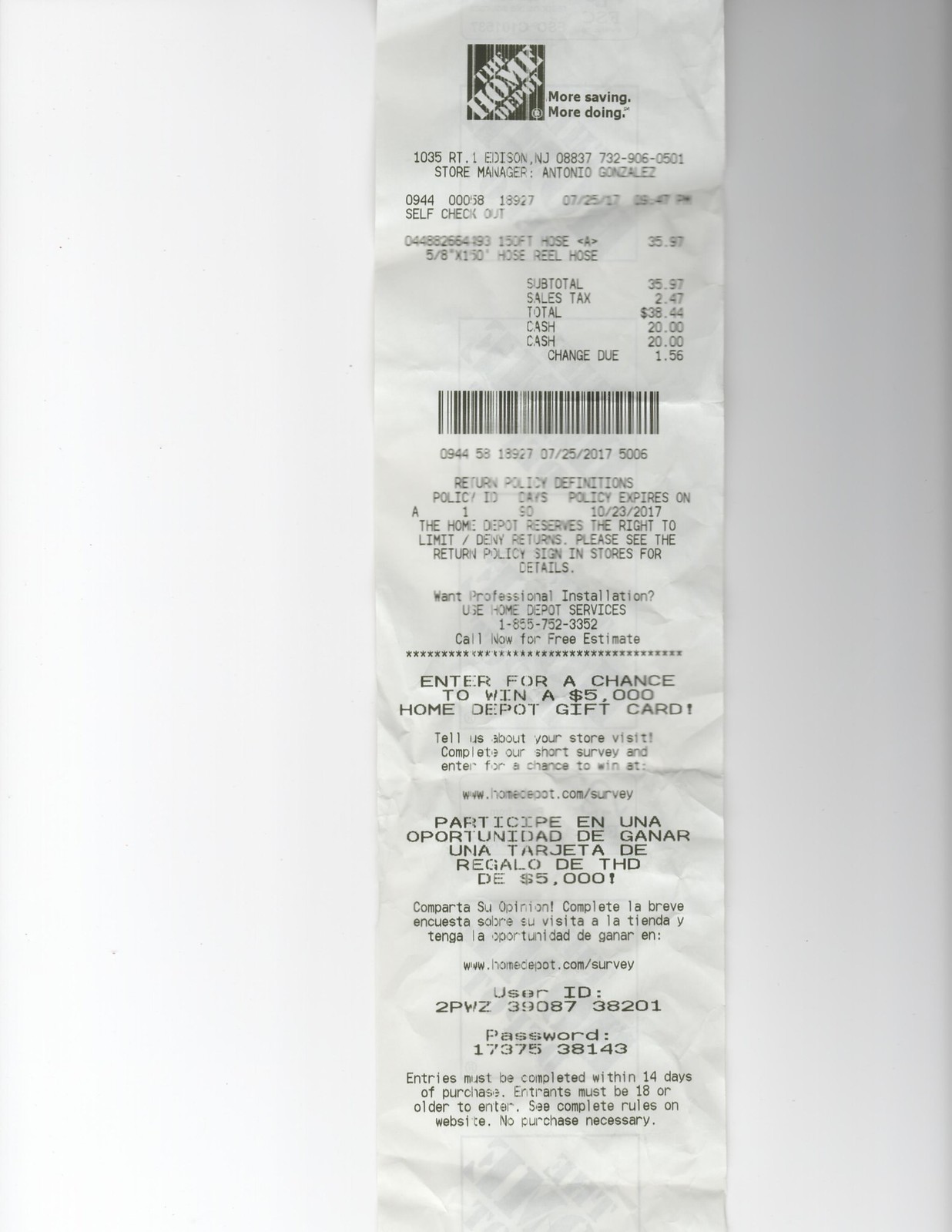The image is an extreme close-up color photograph of a Home Depot receipt placed on a flat, white tabletop. The receipt, slightly crumpled as if it had been stored in a pocket, is made of standard receipt paper with black ink. At the top of the receipt, the Home Depot logo is prominently displayed alongside their slogan, "More Saving, More Doing." This particular transaction took place in Edison, New Jersey, at a self-checkout register managed by Antonio Gonzalez. The purchase was made on July 25th, 2017, at 9:47 PM, for a single item—a hose reel costing $29.97, bringing the total amount to $38.44 after tax. Below the itemized details, there is a barcode and a section on the return policy, which specifies that returns are accepted until October 23, 2017. Further down, the receipt includes information about a survey that offers a chance to win $5,000, with entry details provided in both English and Spanish. The receipt also displays a user ID and password to access the survey.